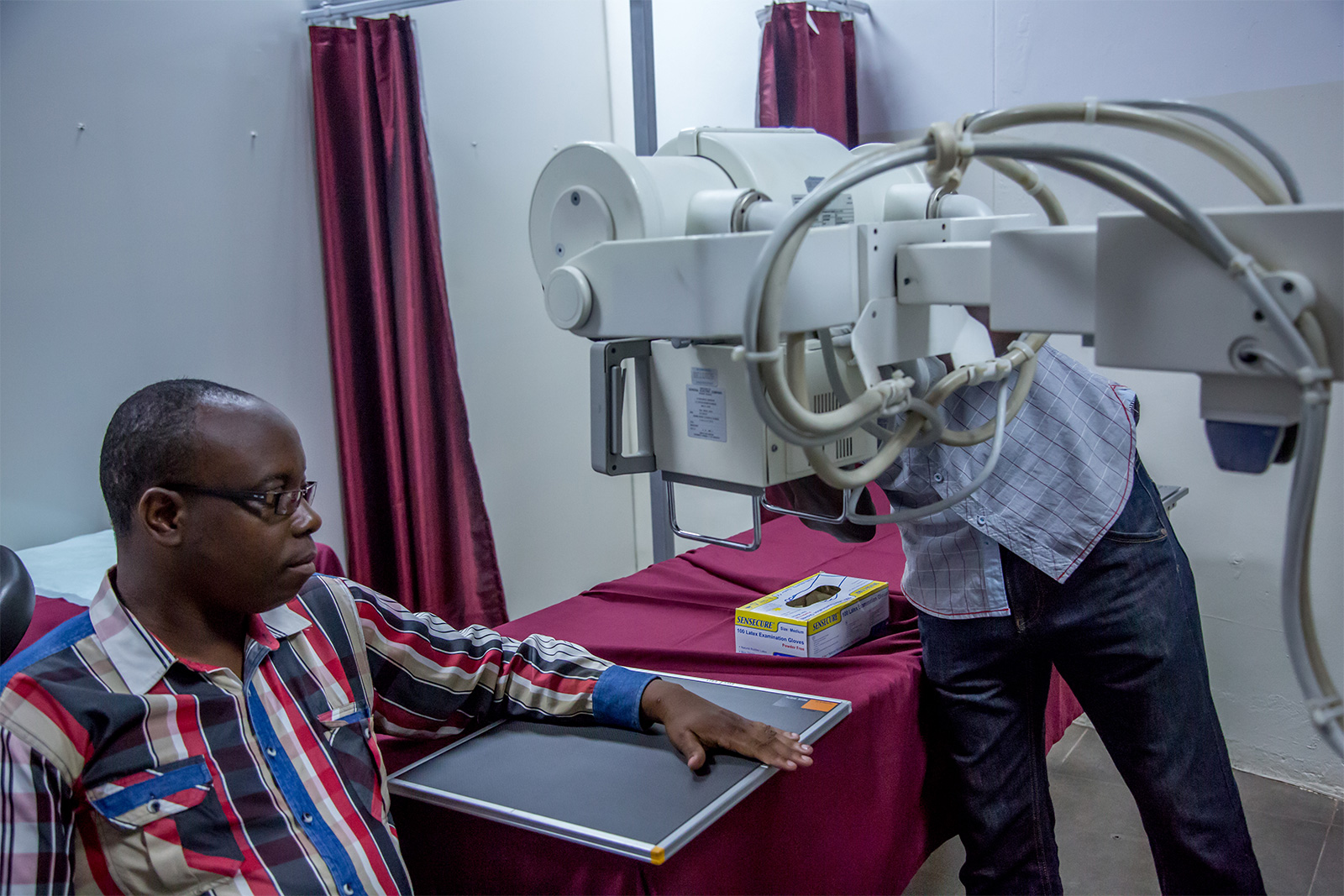In this image, we see a black man with glasses sitting in a chair, wearing a colorful plaid shirt primarily featuring shades of blue, white, and red. His hair is balding at the front. He has his left arm resting flat on a charcoal gray rectangular mat, possibly for a medical procedure. A second person, dressed in blue jeans and a light blue plaid shirt, is standing and manipulating a light gray medical imaging machine equipped with various wires and hoses. This machine appears to be positioned over the seated man's hand, likely conducting some form of scan. The setting is a medical office with a variety of details including a white wall, a magenta privacy curtain, a table covered with a red cloth, and a box of rubber gloves. The room features a gray carpet and is filled with colors such as blue, tan, red, gray, black, silver, and white.